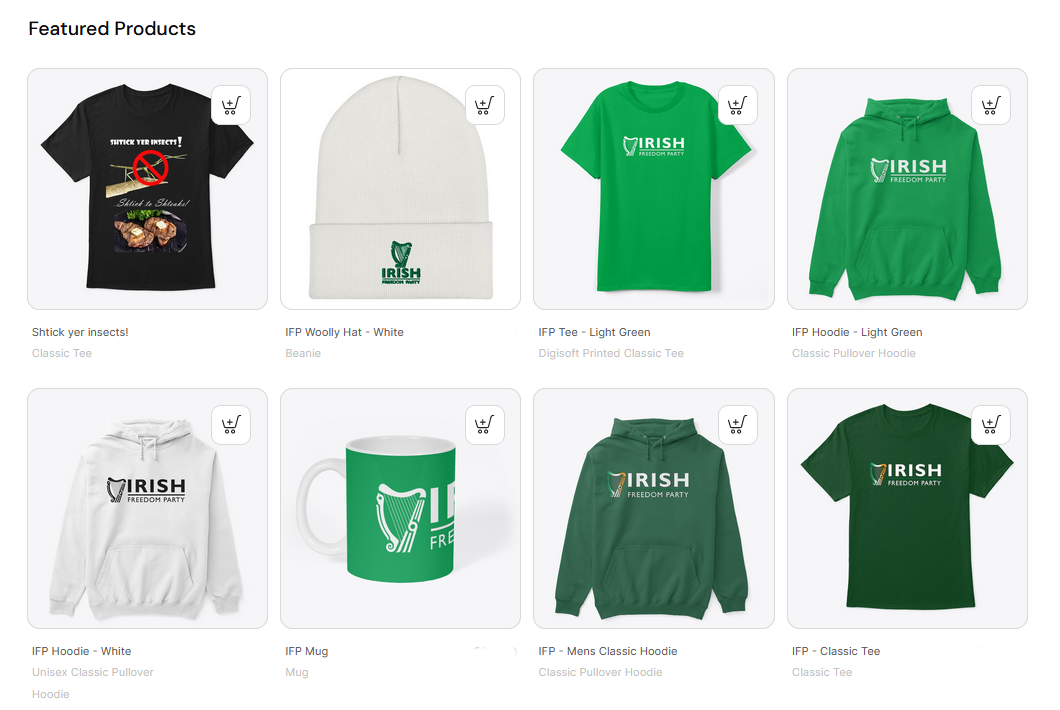This screenshot showcases the "Featured Products" section from a website, clearly labelled at the top left corner in bold black text. The layout consists of two rows, each containing four squares with pale grey backgrounds and rounded edges, all set against a clean white site backdrop.

In the top row, the first square on the left features a black t-shirt adorned with a printed design. Next to it, the second square displays a white beanie with an embroidered logo that reads "Irish." Moving to the third square, there is a bright green, round-neck, short-sleeve t-shirt with a white print of a harp and the word "Irish." The last square on the top row presents a long-sleeve pullover hoodie, also featuring a harp and the word "Irish."

In the second row, the first square on the bottom left showcases a white hoodie pullover with the same black print of a harp and the word "Irish." The second square from the left contains a bright green mug with a white handle, featuring a white harp and the word "Irish" printed on it. The third square features a dark grey, long-sleeve pullover hoodie with a colorful harp and the word "Irish" in white. The final square on the bottom right displays a dark green, round-neck, short-sleeve t-shirt, also adorned with a colorful harp and the word "Irish" in white.